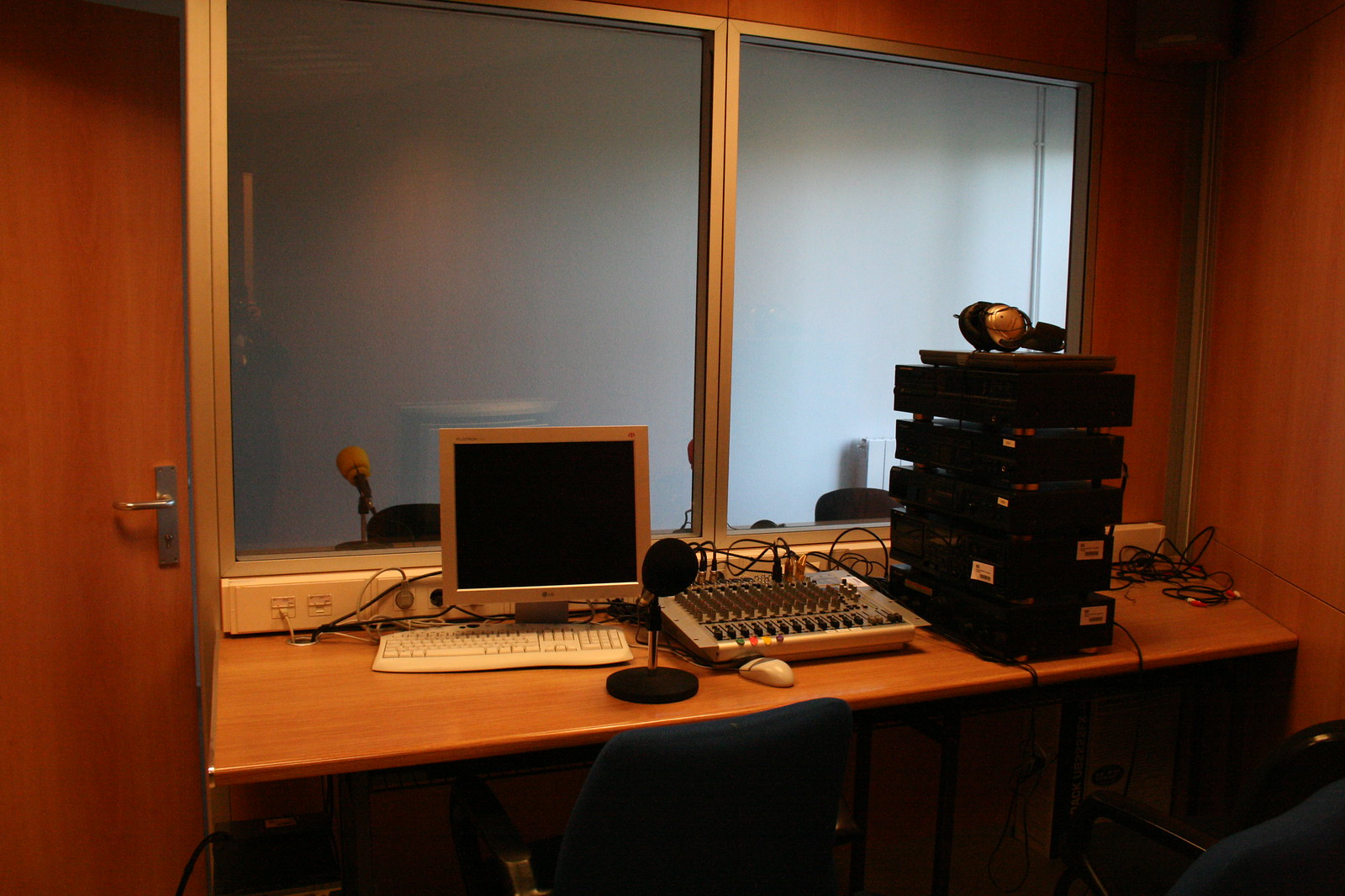This image depicts a small, well-equipped recording studio. The room is furnished with wood elements, including a rust-colored door with a silver handle on the left. In the foreground, a wooden desk is prominently featured, with a black computer monitor, keyboard, and a white mouse. A black microphone and an electronic sound machine with numerous cords and knobs are also present on the desk, along with a stack of rectangular black boxes, atop which rests a pair of predominantly black over-the-ear headphones with one gold ear. To the right, partially visible, is a chair illuminated by a light shining down on the desk. A sliding glass window separates this area from another part of the room, which contains a microphone and two chairs against a white wall. Additionally, various wires are scattered around the desk, some connected to a visible white power strip below the window. The overall impression is of a compact and functional studio space designed for audio recording and production.